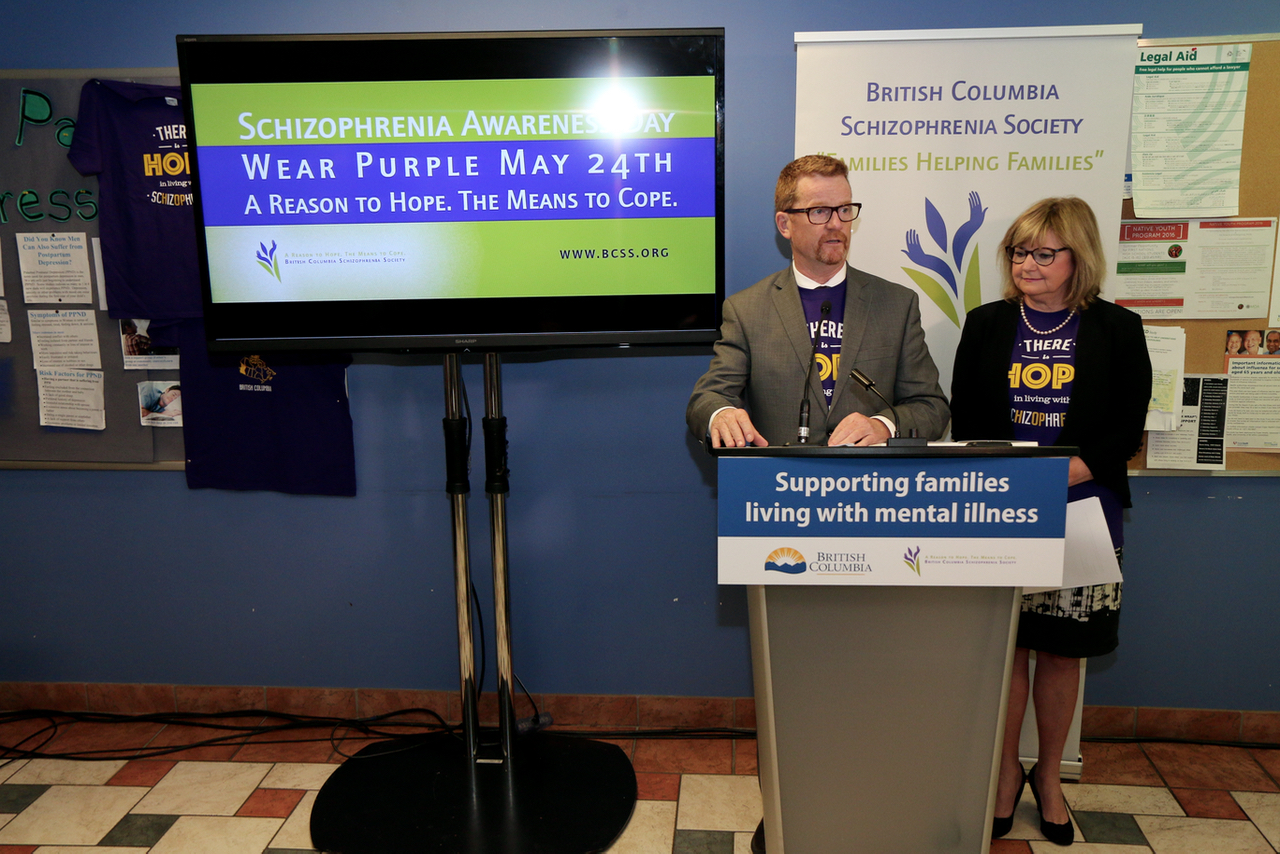In this detailed photograph, a man and a woman stand behind a grey podium at an event hosted by the British Columbia Schizophrenia Society. The man, positioned on the left, has red hair, glasses, and a red beard. He wears a grey suit jacket over a blue British Columbia Schizophrenia Society shirt. The woman next to him has dirty blonde hair, black glasses, and wears a similar blue shirt under a black cardigan, paired with a black skirt and black heels.

To the left of the speakers, there's a mounted television on long silver legs with a black base, displaying a logo on a green background with a purple banner that reads, "Schizophrenia Awareness Day, wear purple, May 24th, a reason to hope, the means to cope." The website www.bcss.org is listed in the bottom right corner of the screen. Left to this television, a board—likely a bulletin or cork board—displays t-shirts and pieces of paper.

The wall behind the podium and television is a calm blue color. Behind the speakers, another bulletin board is visible, covered with various items. The podium itself prominently features a sign on the front that states, "Supporting families living with mental illness." They stand on a colorful tiled floor, suggesting a vibrant and engaging venue for this important awareness event.